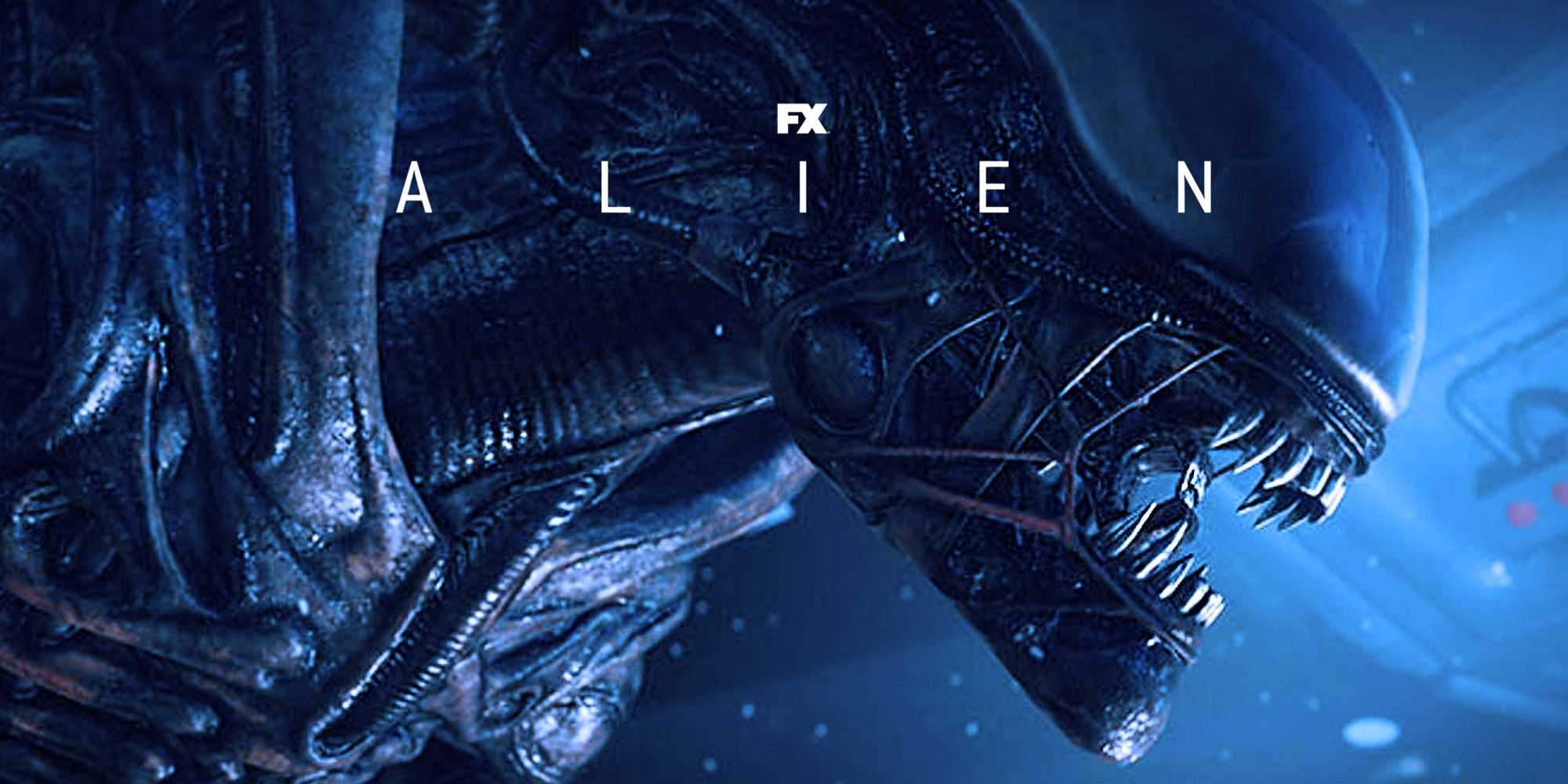This is a highly detailed and atmospheric advertisement for the movie "Alien" on FX. The image is in a widescreen horizontal format and features a close-up of the iconic alien creature from the film. The FX logo is placed centrally at the top in a small font. Directly below it, the word "ALIEN" is spelled out, with letters spaced apart and rendered in white.

The backdrop of the image is a dark, almost ominous blue, mimicking the vast emptiness of space. The alien dominates the frame, with its menacing, elongated head resembling a grotesque helmet and its body displaying a biomechanical exoskeleton. The creature is facing to the right, its mouth agape to reveal razor-sharp teeth, adding to the chilling quality of the scene. 

In the background, there is a hint of a control panel, adorned with a couple of red buttons, suggesting that the event is taking place aboard a spaceship. The overall dark blue tones, coupled with the eerily lit alien, create a deeply unsettling atmosphere, perfectly capturing the horror essence of the movie.